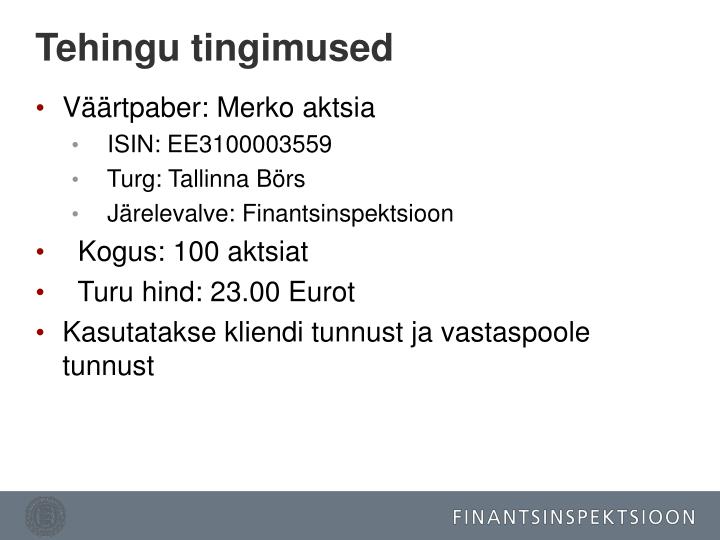The image displays a document against a white background, with text written in a foreign language, presumably Scandinavian. At the top left, the bold black title reads "Tehingu Tingimused." Below the title are four primary red bullet points:

1. **Vartpeber: Merko Actesia**
    - Sub-bullets:
        - **ISIN: EE3100003559**
        - **Terg: Talena Bors**
        - **Jarelevalv: Finansinspektion**
2. **Kogus: 100 Axiat**
3. **Teru Hind: 23.00 Euro**
4. **Kasutaski Kliendi Tunust Ja Vastaspul Tunust**

At the bottom of the page, there's a dark gray rectangle featuring the text "FINANTSINSPEKTSIOON" in white letters positioned on the lower right side.